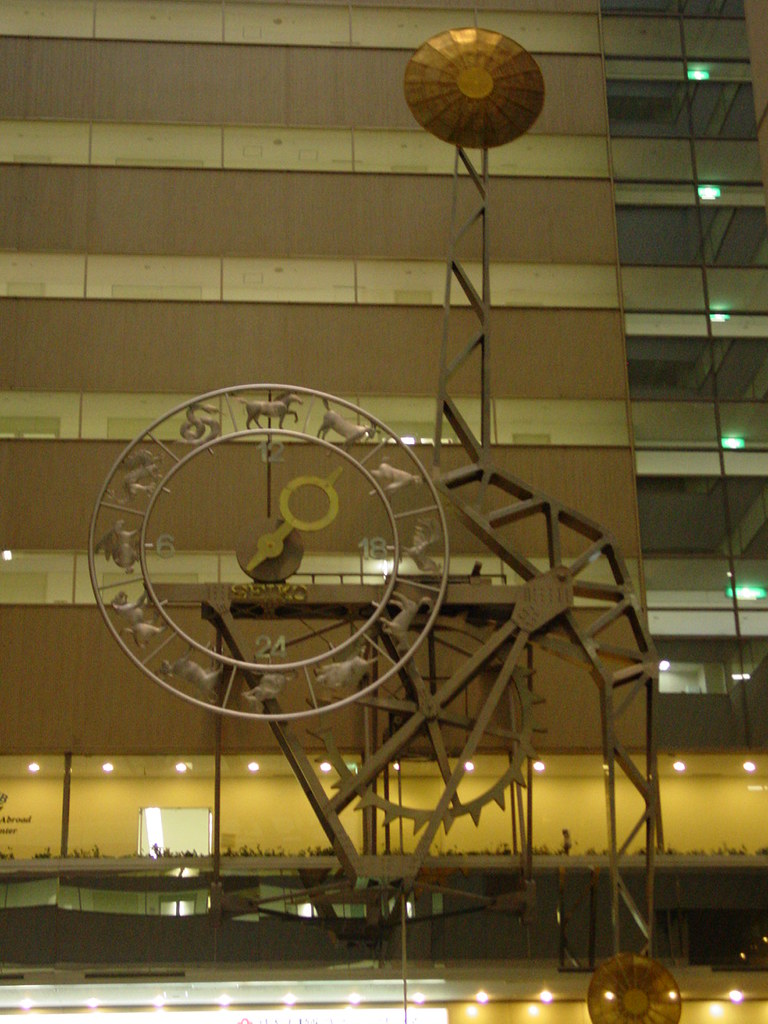The photograph showcases a striking metal sculpture resembling a piece of machinery, prominently positioned in front of a tall, multistory building. The building, which forms the backdrop, features a brown and white façade adorned with numerous windows, some of which are illuminated on the lower levels. The sculpture itself commands attention with its intricate design centered around a large circular dial reminiscent of a clock. Unlike conventional clocks, this dial uniquely displays a series of animal figures in place of the usual numeric markers. Additionally, instead of the standard 12-hour cycle, the dial is marked with the numbers 12, 18, 24, and 6, adding to its unconventional and intriguing appearance. The interplay between the modern industrial aesthetic of the sculpture and the architectural backdrop of the building creates a captivating visual contrast.